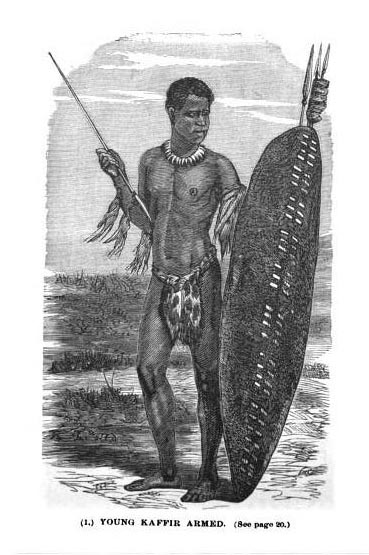In this rectangular black-and-white illustration, likely from a book or museum reference, a young male, possibly of African or Native descent, is depicted standing on a flat, dirt surface. The caption at the bottom of the image reads: "[number one] Young Kafir Armed. [see page 20]." The boy is dark-skinned with short hair, and wears only a loincloth made of a fabric with a jute-like appearance. Around his neck is a necklace, possibly made of teeth or shells, and his arms are adorned with bunched-up material resembling grass. He is shirtless and barefoot. In his right hand, he holds a scepter or spear, and in his left, he clutches a long, dark shield that stretches from his feet to nearly his chin. The shield features a central line with two white patches on either side. The background appears to be a savannah with sparse grass.